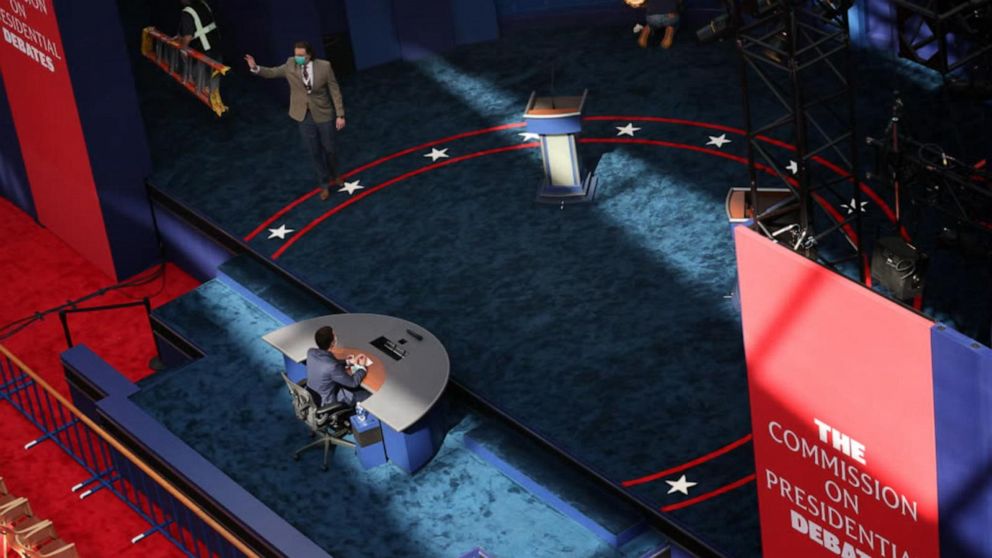The image depicts a top-level view of a debate stage adorned with blue carpeting. Central to the stage is a red semicircle with white stars, bordered by the same blue hue as the carpet. At the lower level, which also features blue carpeting, a person is seated at a semicircular table. This individual, a male with dark hair, wears a blue jacket and faces another person on stage. On the main stage, to the left from the audience's perspective, stands a person in a brown suit jacket and blue pants, waving with their right hand while wearing a light blue mask. Exiting the stage is another individual carrying a ladder. There's a podium with a brown top, matching the stage's blue and white color scheme. In the background, a red carpet and a protective fence are visible, segregating the stage from another area. The words "The Commission on Presidential Debates" are prominently displayed in white on red and blue banners located at both the bottom right and top left of the image.